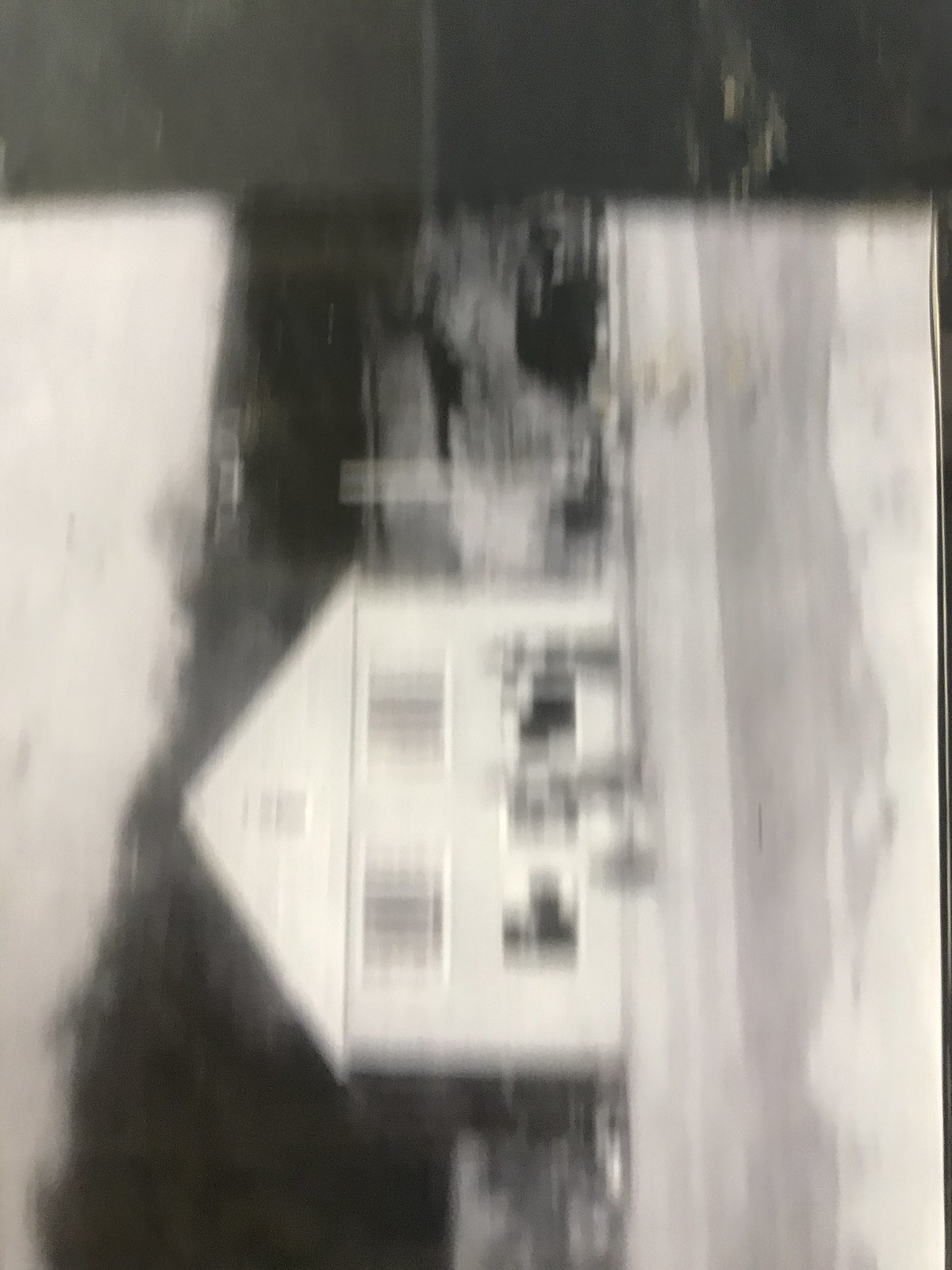The image is a sideways, blurry black-and-white photograph of the front side of a two-story house. To properly view the picture, you would need to turn your head to the left. The ground in front of the house exhibits a gradient of shades, transitioning from light gray to white, then blending into gray, and finally back to light gray.

The house itself is light gray and features two windows. A black car is parked in the driveway to the right of the house. In the backdrop, a clump of trees creates a dark, leafy background that contrasts with the lighter-colored sky above, which appears light gray. At the very top of the image, from this perspective, a dark gray background can be seen.